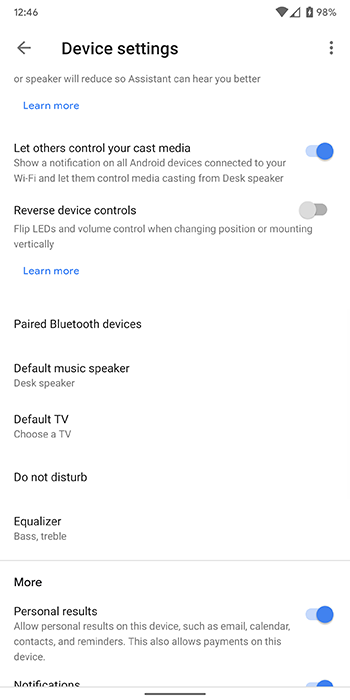A person navigates through the "Device Settings" menu on their Android phone. The screen displays various options that can be adjusted or toggled. 

- **Let others control your cast media**: This feature is turned on, allowing notifications to appear on all Android devices connected to the same Wi-Fi, permitting media control from the desk speaker.
- **Reverse device controls**: This setting is off. It allows the flipping of LEDs and volume control when the device's position is changed or mounted vertically.
- **Prepare Bluetooth devices**: Requires user interaction to manage paired devices.
- **Default music speaker**: Currently set to "Desk Speaker."
- **Default TV**: No TV has been set yet, and this option needs to be selected.
- **Do Not Disturb**: Clicking on this option provides additional customization settings.
- **Equalizer**: Set to emphasize both bass and treble, likely forming a V-shaped audio profile.
- **More, Personal results**: This option is turned on, enabling personal results on the device.
- **Show notifications**: This is also toggled on.

The interface features a white background with predominantly black text, interspersed with a few blue elements for highlights and interactive components. The settings suggest a high level of control and customization over media and device interactions, assuming a connection over a Wi-Fi network.